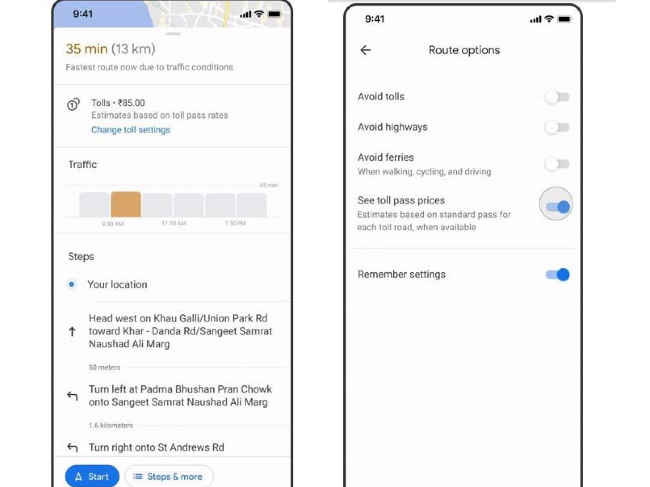---

**Detailed Caption:**

The image features two side-by-side screenshots of a smartphone's interface, showing a navigation app with various details:

### Left Screenshot:

1. **Top Bar:** 
   - Time display: "9:41" in black text inside a blue rectangle with an angled edge covering about one-quarter of the way.
   - Signal strength: Four or five bars displayed as a mushroom-shaped icon.
   - Battery indicator: Shown in black. 

2. **First Section:**
   - Background: Depicts a map with white streets on a gray background.
   - Route Information: "35 MIN" in black text on a yellow background, followed by "(13 KM)".
   - Indicator: A small gray line to the right angled off the parentheses.

3. **Fastest Route Message:** 
   - Text: "Fastest route now due to traffic conditions" in black text.
   - Separator: A horizontal gray line.

4. **Toll Details:**
   - Circle indicators: Two stacked circles with "1" in the top circle next to "Tolls - 85.00".
   - Additional Info: "Estimates based on toll pass rates" in gray text.
   - Button: "Change toll settings" in blue text.

5. **Traffic Information:**
   - Text: "Traffic" with a capital T.
   - Six gray-bordered boxes: The second box is colored tan with inscriptions underneath them.

6. **Steps and Location:**
   - Text: "Steps" with a capital S followed by a blue bullet point and "Your location".

7. **Navigation Instructions:**
   - Direction: A black arrow pointing up.
   - Text: "Head west on Khao Galli / Union Park Rd toward Khar-Danda Rd / Sgt. Samarat."

8. **Additional Directions:**
   - Instruction: "Turn left at Padema Brochure Print Shop onto Sgt. Semrel Neshewed Ali Marg."
   - Distance: "1.6 KM" followed by another direction "Turn right onto St. Andrews Rd."

9. **Start Navigation Button:**
   - Blue oval with a white triangle and "Start".
   - Another oval with "Stops & More".

### Right Screenshot:

1. **Top Bar:** 
   - Similar to the left screenshot with "9:41", signal bars, and battery icon.

2. **Route Options Section:**
   - Arrow pointing left with "Route options".
   - Options: 
     - "Avoid tolls" with a gray toggle button.
     - "Avoid highways" with a gray toggle button.
     - "Avoid ferries" with a gray toggle button.

3. **Additional Details:**
   - Text: "See toll pass prices" followed by gray text mentioning standard pass estimates.

4. **Remember Settings:**
   - Text: "Remember settings".
   - Slider: Light blue area with a blue circle on the right.

Both screenshots are bordered by a black outline on the sides and top. The right screenshot has a predominantly white background.